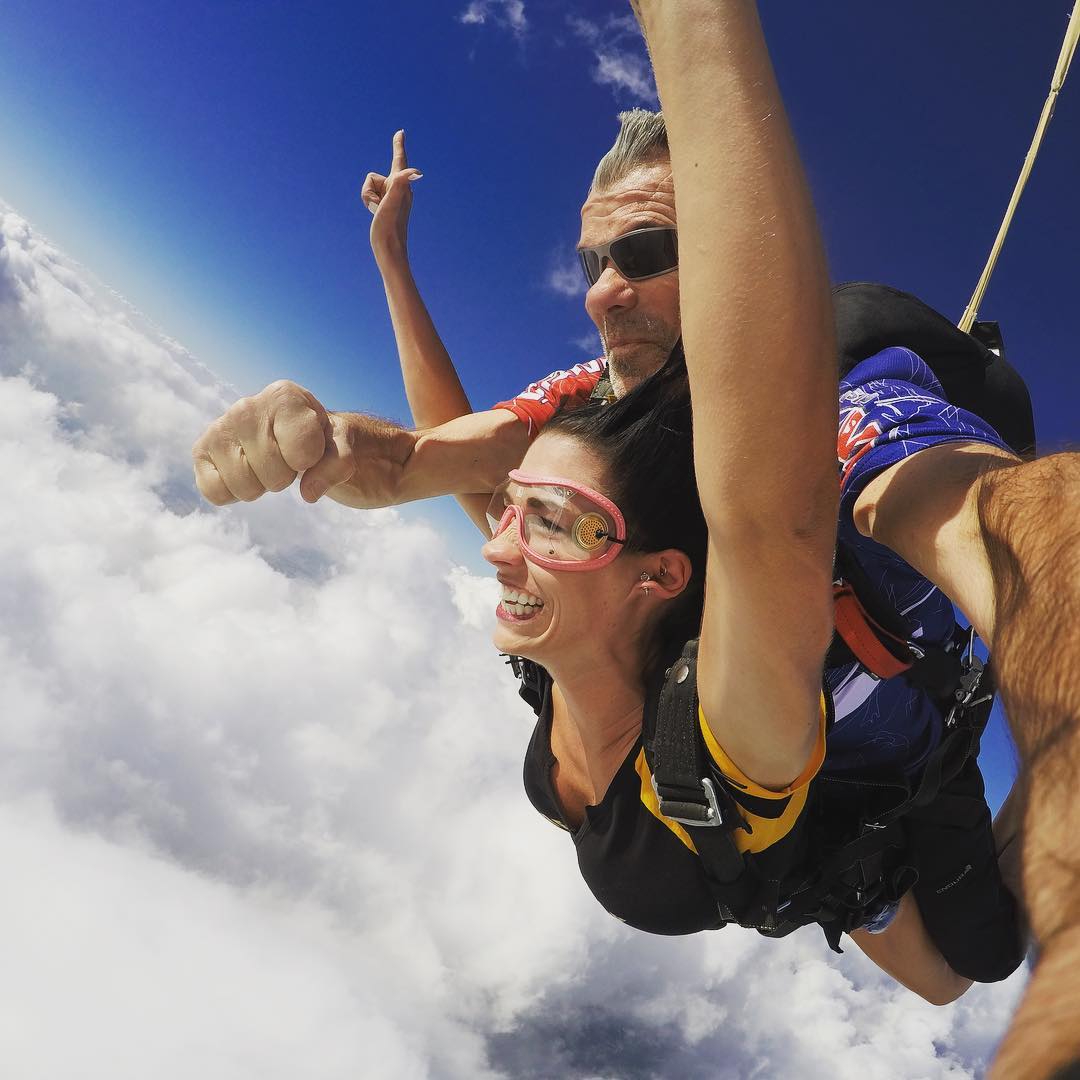In the image, two individuals are captured in the thrilling moment of skydiving, framed by a clear blue sky above and clouds below. The male skydiving instructor, positioned at the top, sports black sunglasses with a gray outline and gray hair. His white face shows a composed expression. Below him, securely attached via parachute straps, is a woman in her 20s or 30s, wearing pink goggles. She is smiling and appears to be filled with a mix of excitement and exhilaration. Dressed in a black and yellow outfit, her joy contrasts with the instructor's calm demeanor. Together, they form a striking image of adventure and the shared human experience of pushing boundaries.